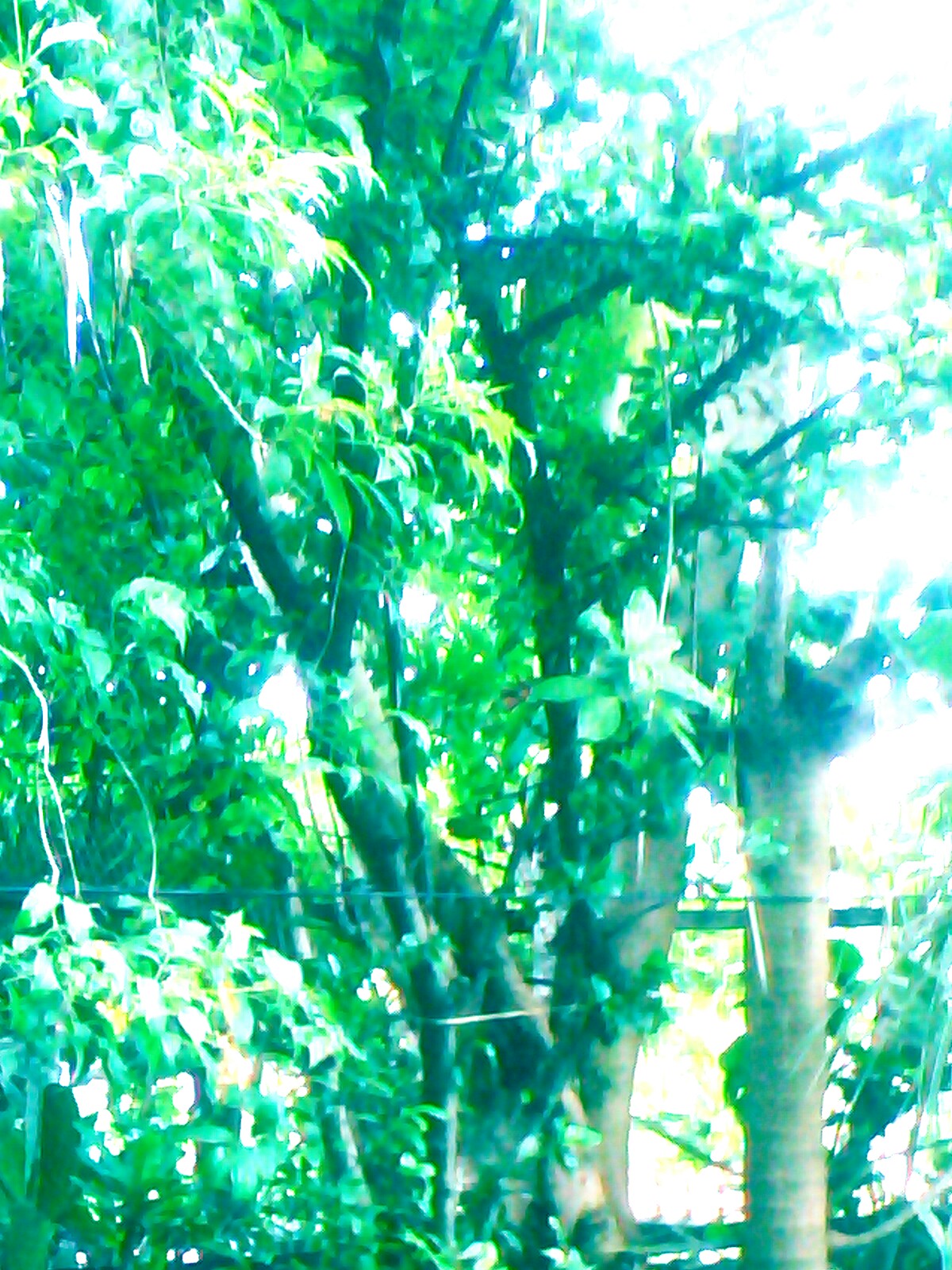The image captures a vibrant outdoor scene brimming with lush green shrubbery and trees, as if you're immersed in a jungle. The bright, sunny day highlights the dense foliage, making the various shades of green leaves and tree branches gleam. Despite a slight blur, the photo clearly shows thick, verdant leaves and limbs intertwining throughout the scene. Towards the lower third of the image, a green wire or bar cuts across, with another thicker, darker green bar or fence visible further in the background.

On the right-hand side, sunlight pierces through the branches, making the foliage glimmer with hints of white and pink, while the left-hand side showcases a mix of light and dark green leaves. The lighting gradient creates a striking contrast, making the upper and right portions of the picture much brighter compared to the darker lower sections. A tree trunk emerges from the lower right, adding to the scene’s lushness, alongside potentially other vegetation like bushes, although the dense foliage makes distinguishing individual plants somewhat challenging. Overall, the image is a beautifully lit portrayal of nature's exuberance.